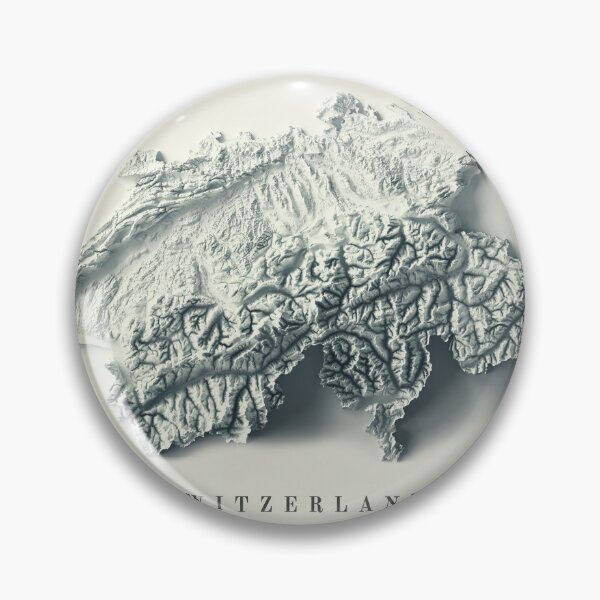The image features a square button set against a white background, designed with a central circular region that resembles a zoomed-in lens view. This lens-like area showcases a topographic, black-and-white representation of Switzerland. Though the entire country is not depicted, the detailed map highlights its mountainous regions with varying shades of gray, adding texture to indicate elevation differences. The outlined mountains appear irregular, almost like brain lobes, with ridges and straight lines scattered across the bottom. On the bottom edge of the button, the word "Switzerland" is partially visible in black text, though the S, W, and D, along with part of the N, are cut off due to the button's edge.